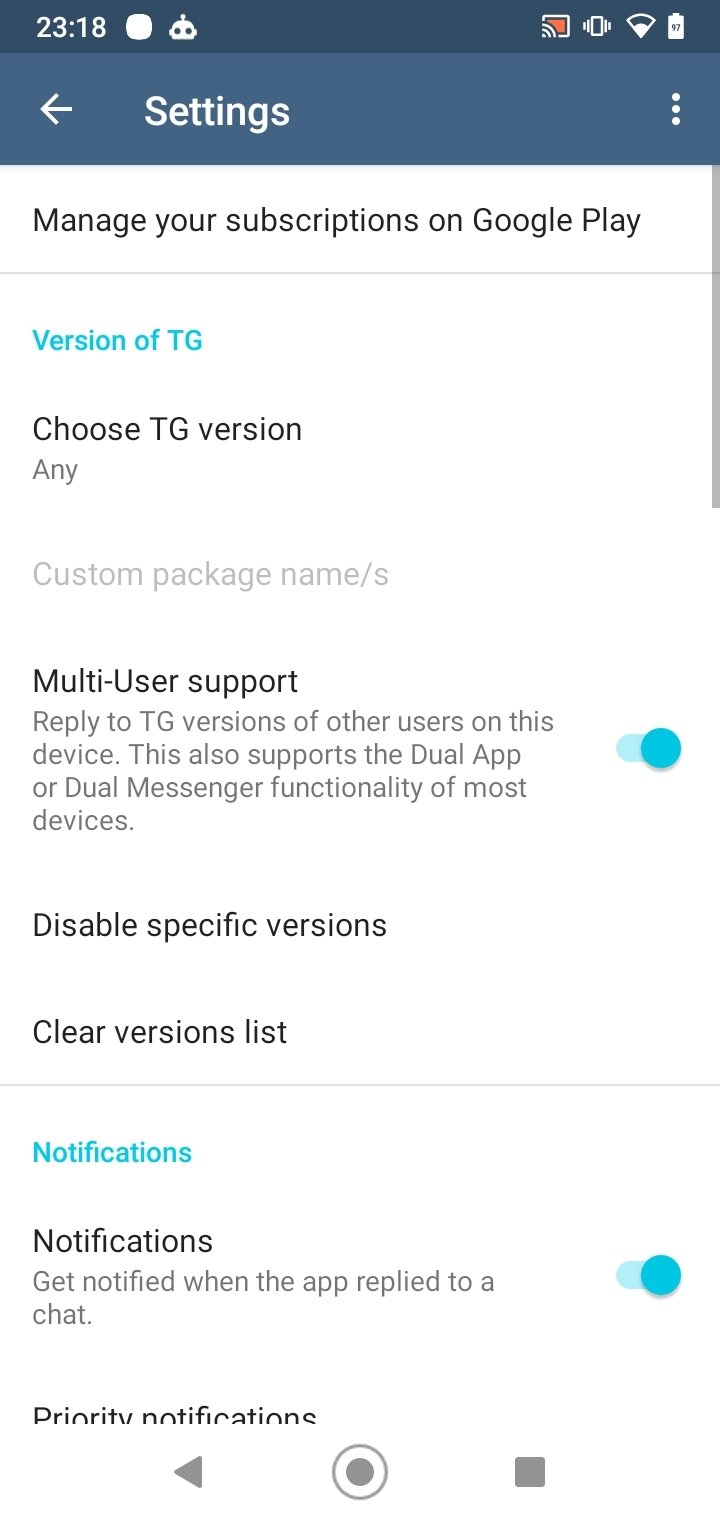Screenshot Description: Google Play Settings Page

The screenshot showcases the "Settings" page of a telephone's Google Play app. At the top, an aqua-colored box displays the title "Settings," with a left-pointing arrow on the left side and three vertical dots on the right side, indicating additional options.

Below this header, the background transitions to white. The first item listed is "Manage subscriptions on Google Play." Following this, in aqua text, the phrase "Version of TG" is visible, accompanied by "Choose TG version" below it.

Subsequently, the "Multi-user support" section is shown. This section instructs users to "Reply to TG versions of other users on this device" and highlights that it supports dual app or dual messenger functionality available on most devices. An aqua-colored toggle button indicates that this feature is activated.

The next options listed are "Disable specific versions" and "Clear versions list," followed by the "Notifications" section. Here, the word "Notifications" is highlighted in aqua, with subsequent text in black explaining that users can "Get notified when the app replied to a chat." Another teal button is shown to be in the 'on' position.

At the very base of the screenshot, partial icons of the phone interface for going back, closing, or returning to the home screen are faintly visible.